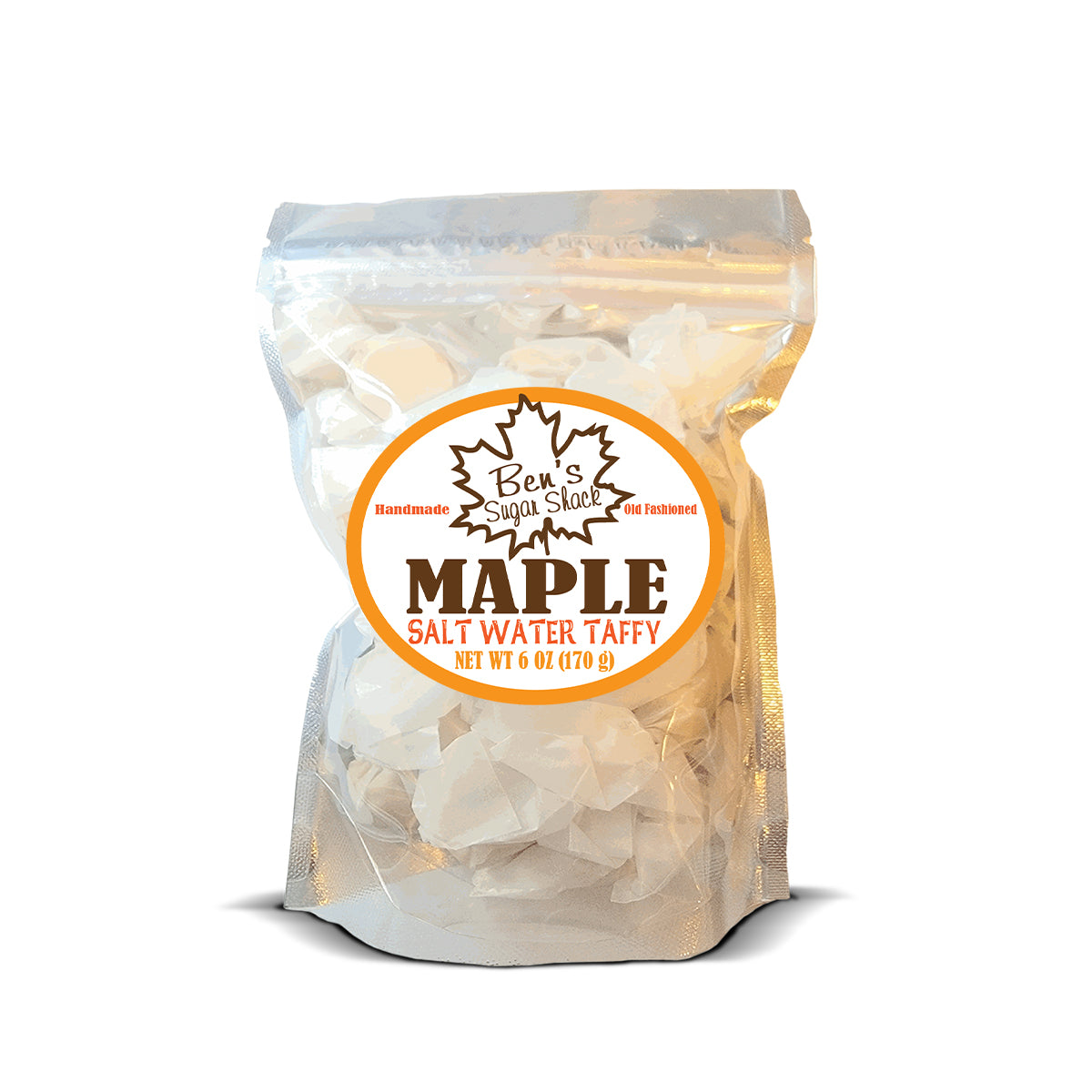The image shows a bag of saltwater taffy, packaged in a silvery bag with clear sections revealing a variety of wrapped taffy pieces inside. The bag, which features a resealable zip-top, stands upright against a white background. Prominently displayed on the front is a label with an orange-edged, yellowish-brown oval design encircling a white maple leaf with the text "Ben's Sugar Shack" in brown. The label also includes the phrases "Handmade" on the left and "Old-Fashioned" on the right. Below the maple leaf, "Maple Saltwater Taffy" is printed in red and brown lettering. The label further notes the net weight as "6 oz (170g)." The taffy pieces inside the bag are individually wrapped in white paper.